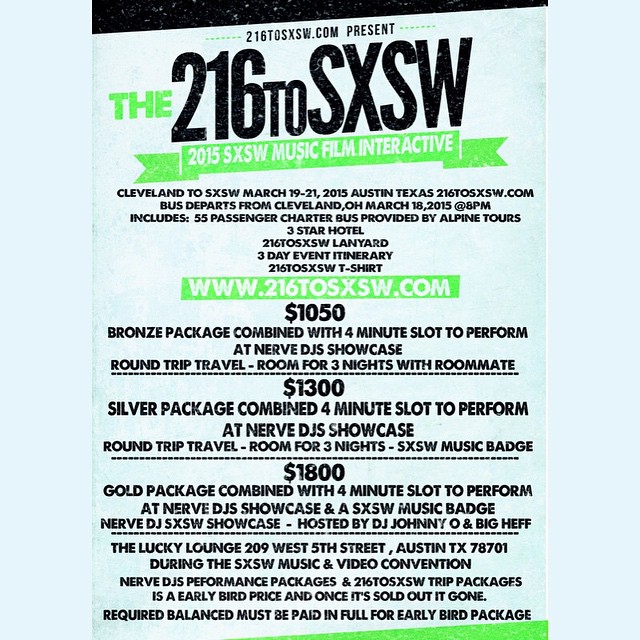The image is a scan or picture of an advertisement poster for the 2015 SXSW Music, Film, and Interactive event, presented by 216TOSXSW.com. The background is primarily light blue and white with sections of green, hosting predominantly black and some green text. The headline at the top reads, "216 to SXSW - The 2015 SXSW Music, Film, Interactive." The event specifics follow with the text, "Cleveland to SXSW, March 19-21, 2015, Austin, Texas." 

The poster details various package options for the trip, including:
- The Bronze Package for $1,050
- The Silver Package for $1,300
- The Gold Package for $1,800

Each package includes a passenger charter bus from Cleveland, a three-star hotel stay, a lanyard, an itinerary, and a t-shirt. At the bottom, the text specifies the address: "The Lucky Lounge, 209 West 5th Street, Austin, Texas" and mentions that the balance must be paid in full for the early bird package.